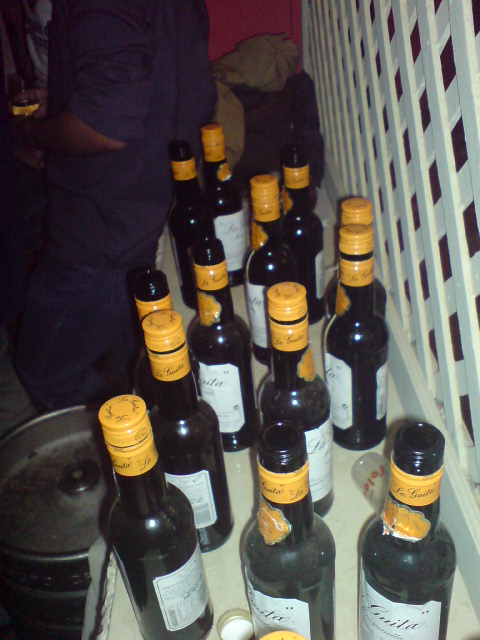This color photograph captures a backyard scene where multiple dark-colored liquor bottles, presumably wine, are aligned on a white surface, which could be a side table or a shelf. Each bottle has a distinct white label and yellow detailing around the cap, with some bottles being open while others remain sealed with their yellow lids. The background features a white trellis fence forming a diamond pattern, partially visible through the lattice design. In the top left corner, a couple of people, one possibly in a blue shirt and jeans, are standing, though their faces are not visible. Additionally, a metal beer keg is seen at the bottom left. The setting suggests a casual outdoor gathering or setup.